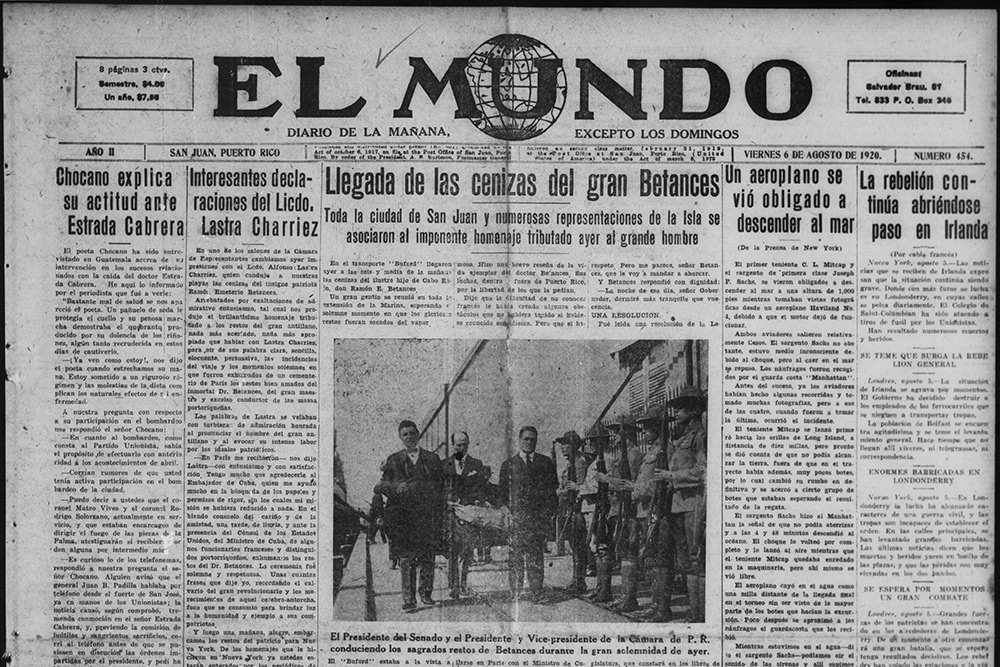This picture showcases an old newspaper, "El Mundo Diario de la Mañana excepto los Domingos," published on Friday, August 6, 1920, in San Juan, Puerto Rico, issue number 454. The newspaper, oriented horizontally, features light gray paper with black ink, entirely written in Spanish. The central headline reads "Llegada de las Cenizas del Gran Betances," and beneath it, an evocative photograph depicts three men in suits—identified as the President of the Senate and the President and Vice President of the Chamber—walking alongside soldiers standing at attention. The article seems to pay tribute to a significant figure, possibly someone who recently passed away. The top right corner of the newspaper includes contact information, such as a telephone number and a P.O. box, hinting at the publication's office. This detailed periodical offers a glimpse into historical events with its meticulous layout and poignant imagery.